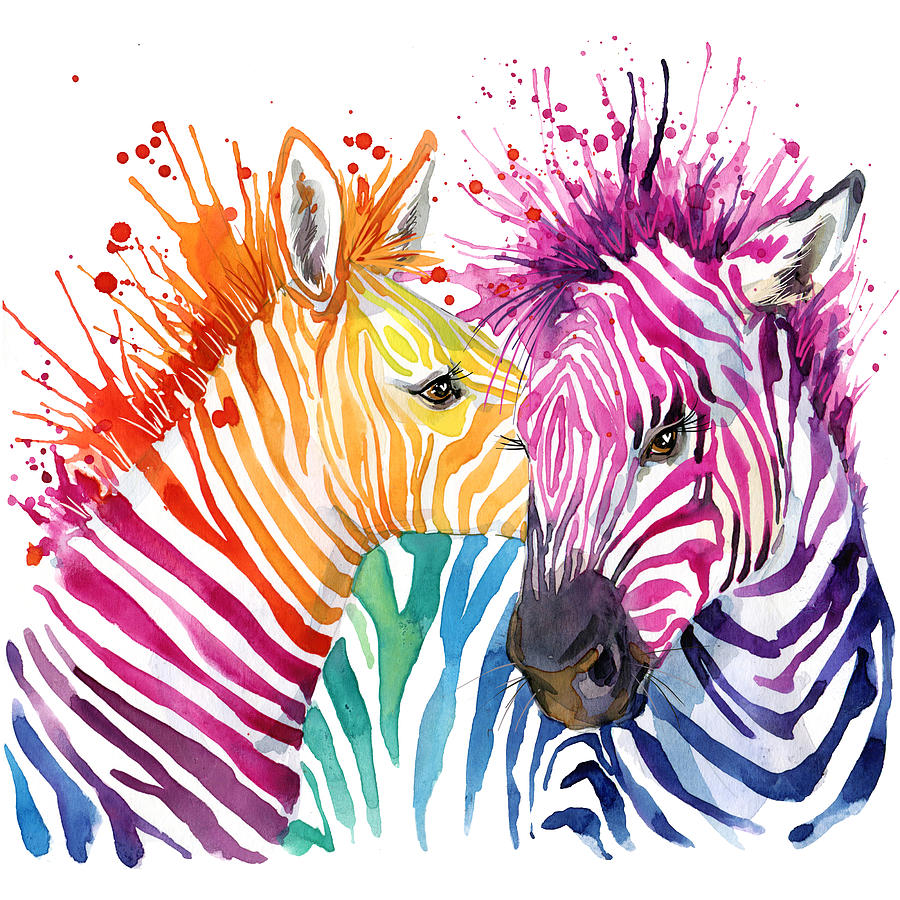This vibrant, contemporary painting showcases two zebras adorned in a stunning array of rainbow colors instead of their traditional black and white. The zebra on the left features a dynamic pattern of yellow, orange, pink, blue, and purple stripes, with orange being the dominant color in its mane dotted with intricate spots. This zebra, which seems to be almost kissing the head of the other zebra, has an eye-catching, detailed appearance, including vibrant eyelashes and visible whiskers on its brown snout. Facing towards the right, the left zebra's profile is highly expressive with wide-open eyes and upright ears. 

Contrastingly, the larger zebra on the right flaunts shades of blue and green with striking pink stripes decorating its face. Its mane, also adorned with dots, enhances the whimsical feel of the painting. The right zebra's colorful display continues the theme of vivid vibrancy found throughout the illustration. Overall, the artwork exudes a joyous, whimsical atmosphere, captivating viewers with its detailed blending of playful colors and meticulous detailing of the zebras' expressions and features.